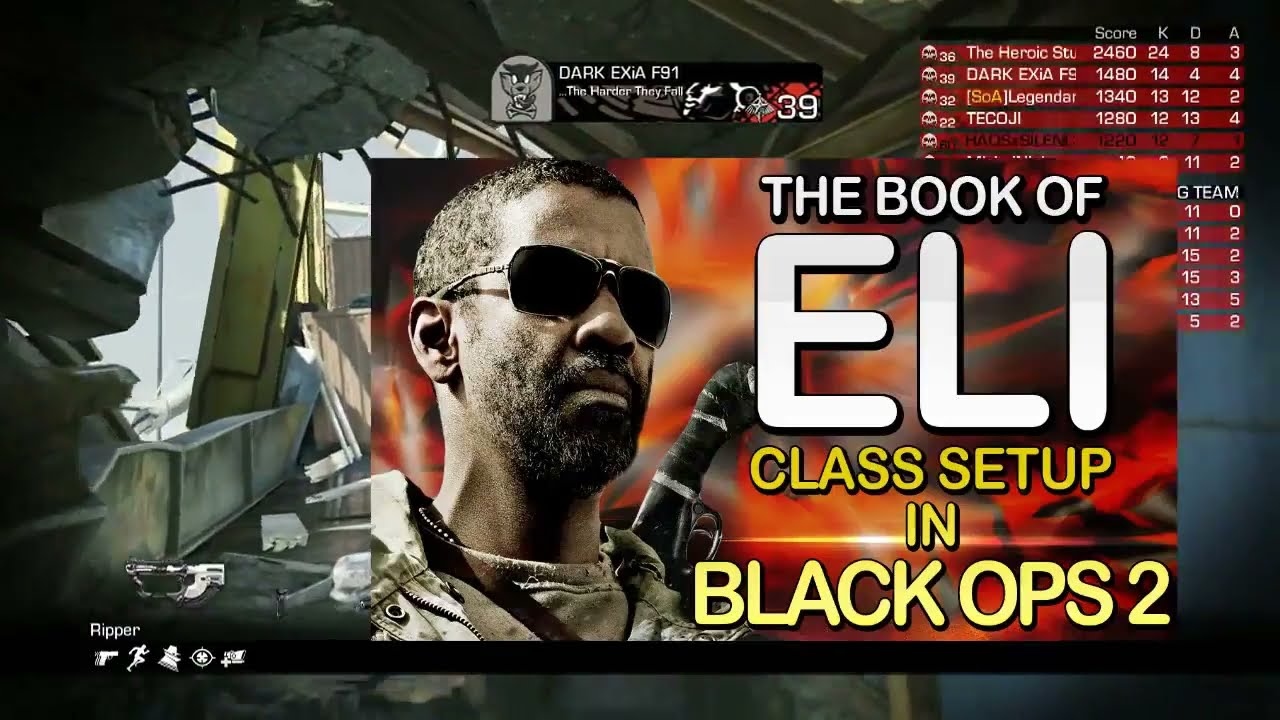The image features a multi-layered design set against a dark background. At the top, in large gray uppercase letters, is the logo "TK," outlined in blue, adjacent to the word "Chaos," also in gray with a blue border. The central focus of the image is a red rectangle, within which Denzel Washington, wearing dark aviator sunglasses and a camouflage jacket, is depicted. Above him, the text "The Book of Eli" is written in white letters framed by a black shadow. Below this, the caption "Class Setup in Black Ops 2" appears in a bold yellow font. A noticeable feature on the left side of the image is two round, white pressed pills with skulls on them, flanked by a gray band labeled "FPS Freak Phantom." Along the bottom of the image is the text "Receive 10% off any Control Freak using code Chaos X Silencer," combining white and green fonts for visual emphasis. The overall color scheme is highlighted by intricate details such as the faint skull-like images that blend into the dark background, adding depth and complexity to the scene.